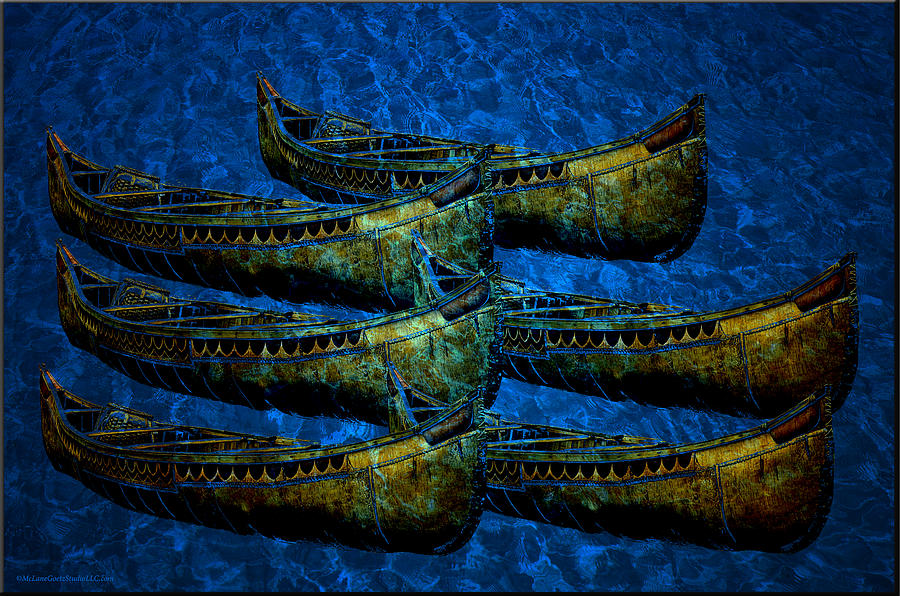This is a detailed and vibrant abstract painting titled "McLean Quits Studios LLC," depicting six canoe-like boats arranged artfully on a blue background that evokes the sense of looking into a swimming pool. The background, with its ripples and variations of clear blue, suggests water but remains distinctly non-realistic. The boats, reminiscent of Viking longships or pirate ships, are positioned with three on the left, two on the right, and one centrally overlapping the others. These vessels are adorned with a rich palette of greens, oranges, reds, browns, and touches of blue, featuring intricate details such as inverted arches of black and small holes along the sides. The overall composition is distinctly artsy, with a slight metallic or worn appearance contributing to its intriguing and visually captivating style.